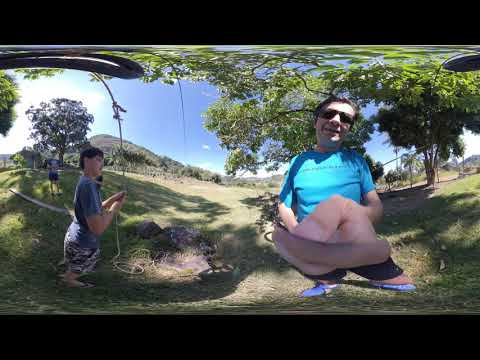The image captures an outdoor scene bathed in sunlight with a blue sky and no clouds in sight, reflecting a serene day. Dominating the foreground is a man seated, clad in a blue t-shirt, black sunglasses, and blue shoes, seemingly holding the camera at arm's length. Beside him to the left is a boy or teenager, dressed in a blue short-sleeved t-shirt and gray-and-white camo shorts, gripping a rope that dangles from a nearby tree with lush green leaves. The reflection reveals a verdant setting of grass and trees, extending to an open hillside in the distance. Although slightly blurred, another boy in similar attire can be glimpsed standing further back, enveloped by the vibrant greenery. The man's camera captures the arc of the trees, adding a dynamic curve to the background and enhancing the sense of depth in this bright, tranquil landscape.